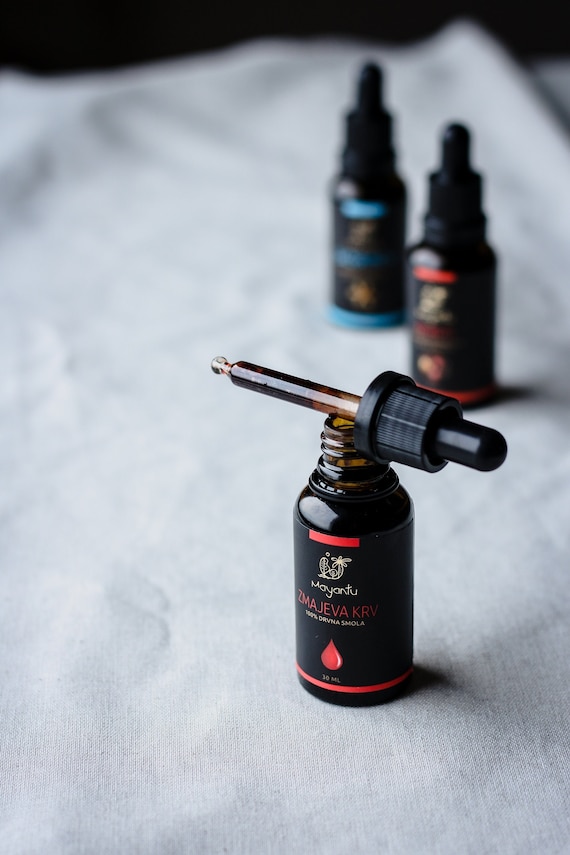This is a detailed close-up photograph focusing on a dark brown bottle with a dropper top prominently situated in the foreground. The dropper, featuring a black squeezer end, is placed horizontally on the open mouth of the bottle. The cylindrical shape of the bottle tapers to a smaller base, indicating it is likely made of glass. The bottle sports a black label adorned with intricate details: a symbol resembling the letter B that transitions into a palm tree, the brand name "Mayantu" in white text, and below it in red, the text "ZMAJEVA KERV". Further down, the label reads "100% DRIVAS MOLLA, DRVETNA SMOLA", with a red teardrop icon and "30 milliliters" in white. Positioned on a gray or white piece of fabric, the scene also includes two additional bottles in the background. These background bottles are blurred; the one on the left has a cyan-tinted label, and the one on the right appears similar in design to the foreground bottle but with a potentially lighter red label. The setting is a well-lit room, sharply drawing attention to the detailed foreground bottle and its dropper apparatus.